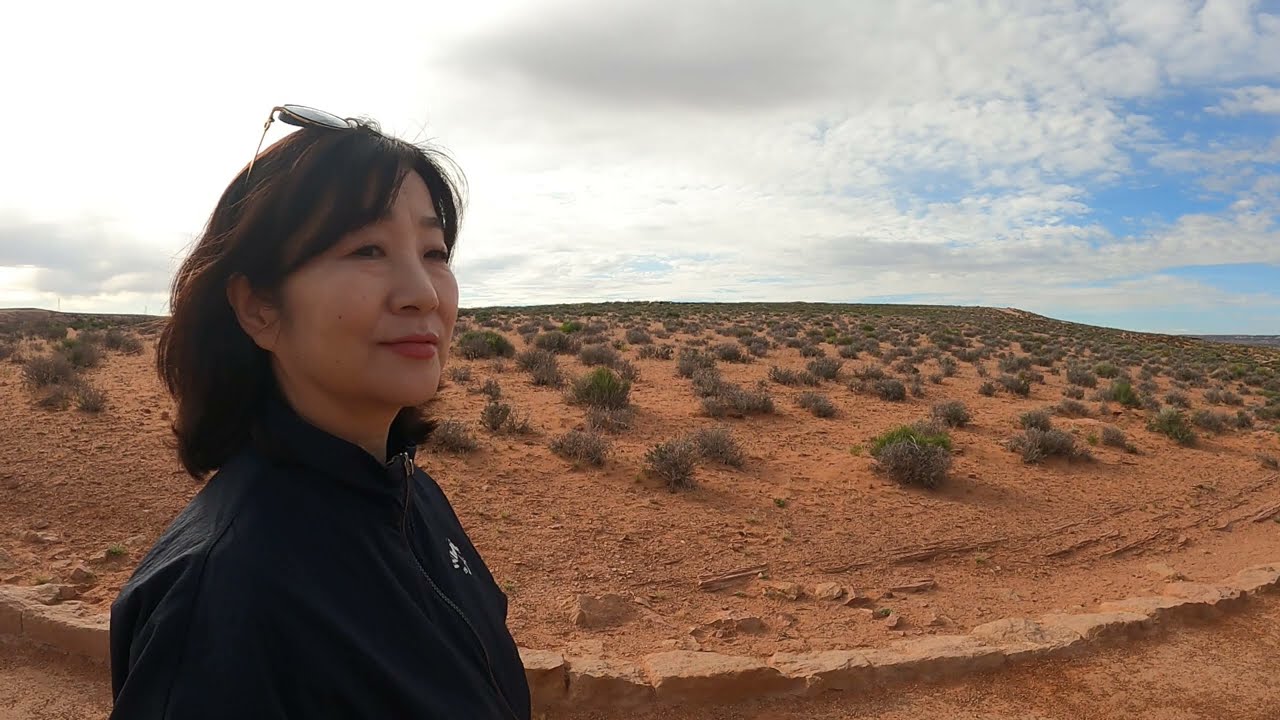The image is a full-color photograph taken outdoors in a desert area on a mostly cloudy day. The sky is predominantly cloudy with patches of blue visible. The ground is a mix of sand, dirt, clay, and sparse scrub bushes, most of which are brown and dry, while some retain a hint of green. The central focus of the image is an Asian woman standing towards the left edge, with her body slightly turned to the right and her head facing the same direction, but not directly at the camera. She has shoulder-length brown hair and is sporting a pair of sunglasses perched on top of her head. She wears a dark blue zip-up windbreaker jacket and has a gentle smile on her face. The backdrop extends to the horizon, illustrating the coarse, arid landscape dotted with dry shrubs.